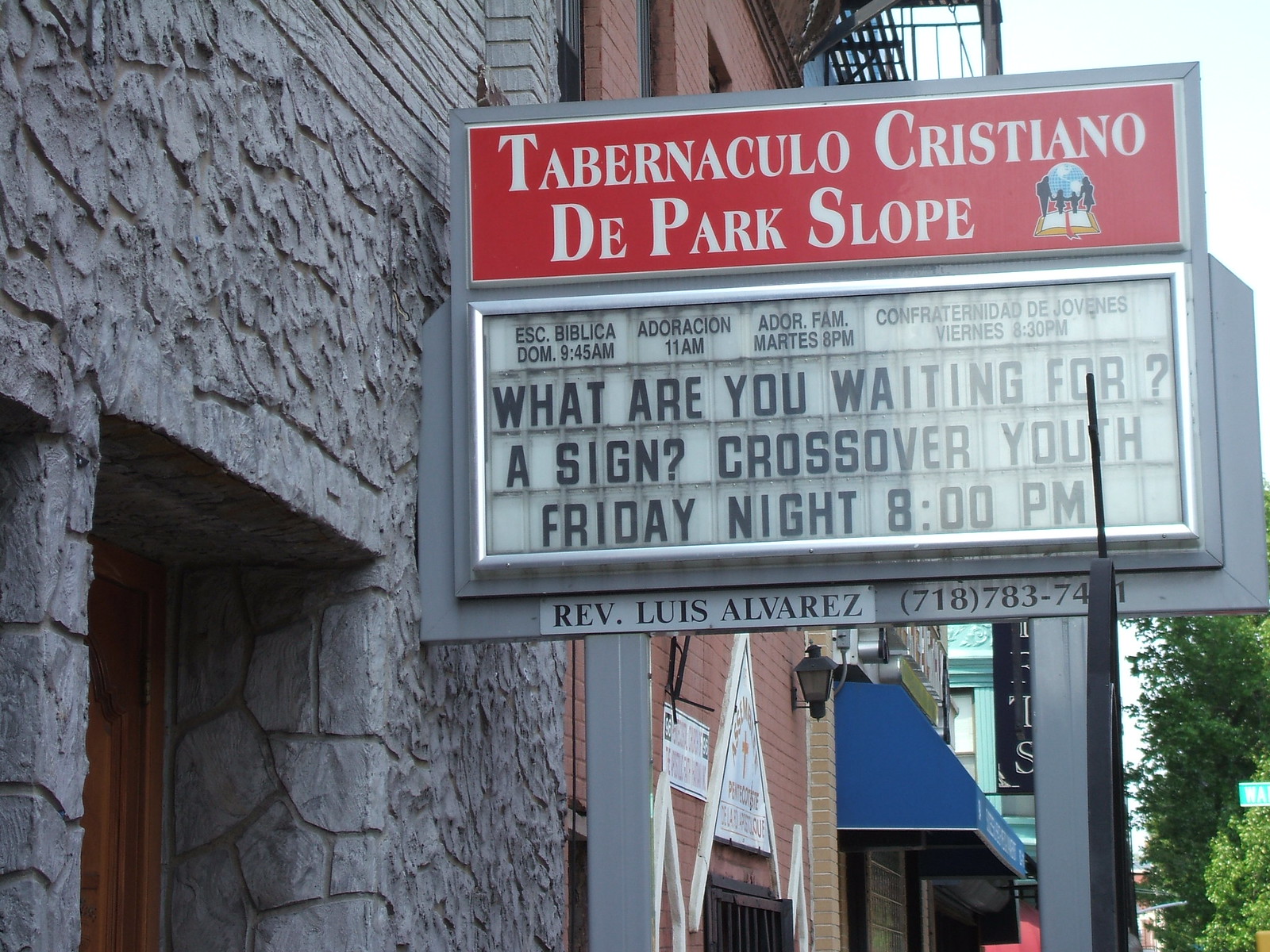The photograph features the front of a building, likely a church known as "Tabernaculo Cristiano de Park Slope." Prominently displayed is an old-fashioned, changeable letter marquee sign typically used for theaters, where someone manually arranges each letter. The sign's top text is in red, reading "Tabernaculo Cristiano de Park Slope," with a silver border surrounding the white letters. Beneath this, in English, it declares, "What are you waiting for? A sign? Crossover Youth, Friday night, 8:00 p.m." Additionally, a sticker banner at the bottom provides the name and contact number of Reverend Luis Alvarez, with the area code 718, indicating a possible South American setting where both Spanish and English are used. Surrounding the focal sign, there are indistinct storefronts and various shops, pointing to the building's location within a mixed-use urban area.